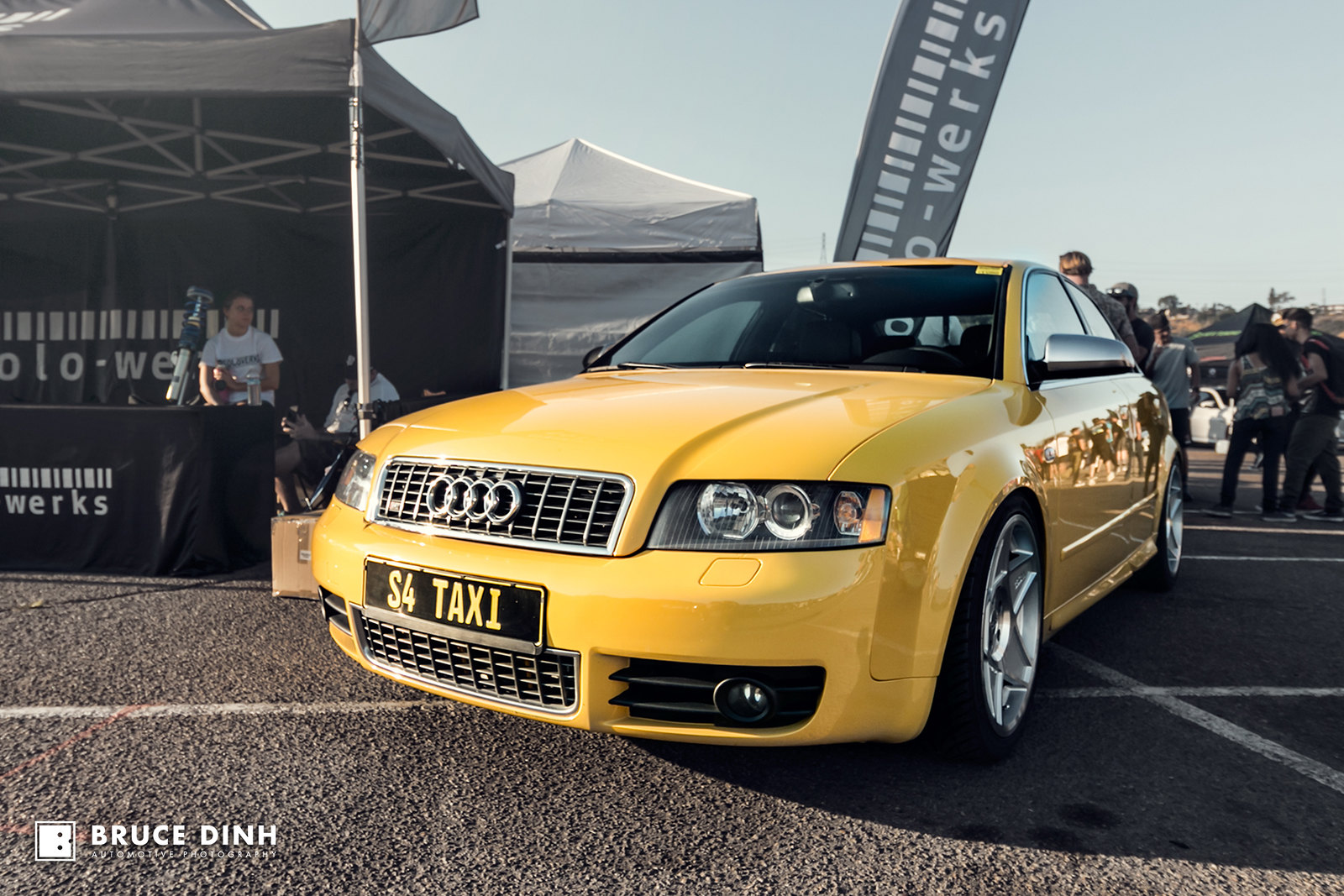This is a detailed photograph of a new and shiny yellow Audi sports car, showcased as a taxi with "S4 Taxi" displayed in gold lettering on a black front license plate. The car is positioned at an angle, offering a clear view of both its front and a portion of its side. It is parked on a ground with white lines that resemble a parking lot. Surrounding the car, there are several people casually standing and interacting, some of whom wear white shirts. Behind the car, we can spot two tents; one black tent to the left, partly obscured by the vehicle, displays the word "WERKS" on its banner, and there is another tent in the background. The sky overhead is light blue, contributing to the bright and vibrant ambiance of the scene. Notably, in the bottom left corner of the image, there is a square logo with "Bruce Dean" written in white on it, adding a subtle branding touch to the photograph.